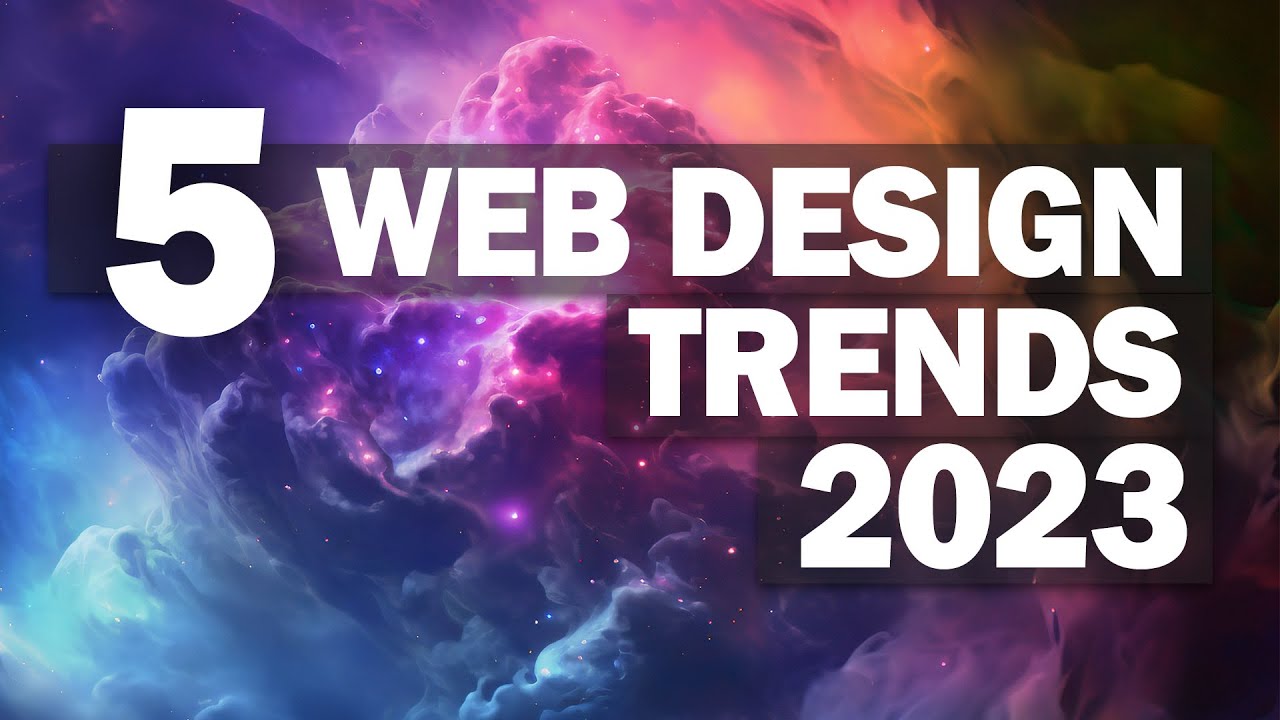In a captivating, horizontally oriented image resembling a video thumbnail, the foreground features bold white lettering that reads, "Five Web Design Trends 2023." A large number "5" dominates the scene, with "web design" written in a slightly smaller script beneath it, followed by "trends" and the year "2023." The background presents an ethereal mix of purple, blue, and lighter pink hues, reminiscent of either large, diffused clouds or a nebula-like cosmic scene, complete with sparkling stars and a science fiction vibe. The contrasting dark elements and vibrant celestial colors evoke the imagery of a distant galaxy, similar to those captured by the Hubble Space Telescope.